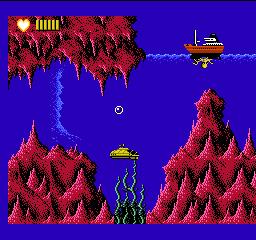The image is a screen grab from a video game, presented in a square format with an overall blue background, suggesting an underwater scene. In the upper right corner, a wavy horizontal lighter blue line hints at the water's surface. Floating on this ripple is a ship. On the upper left, there's a red object resembling an upside-down mountain with pointed tips hanging downward. This shape is mirrored on the bottom left, where a similar red object displays its tips pointing upwards.

At the center-bottom of the image, a few thin strands of seagrass float gracefully upwards. Positioned to the right of the seagrass is a large, towering red structure, reminiscent of an underwater mountain, extending upward. Just above the seagrass, a small yellow submarine is visible, adding a touch of intrigue and exploration to the scene.